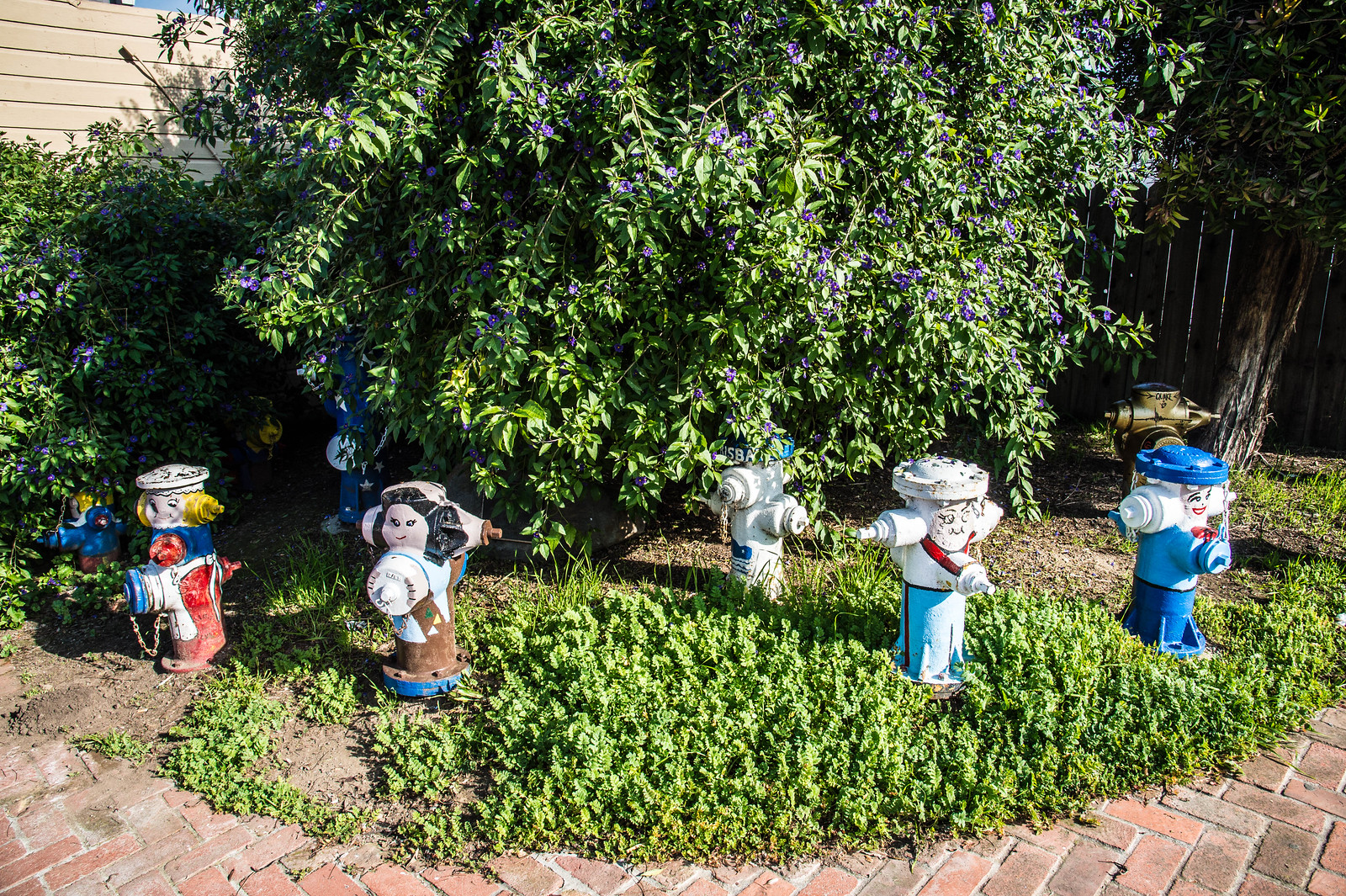This photo captures a whimsical scene in someone's front yard, where six or seven fire hydrants have been creatively transformed to resemble various characters, resembling garden gnomes or cartoon figures. Situated amidst a mix of foliage that includes a lush bush adorned with small purple flowers and a tree, the hydrants display a range of vivid colors and playful designs. 

From left to right, the first hydrant appears half-hidden in the greenery, painted in shades of blue and yellow. The following hydrant is notably decked out with a white face, yellow accents, and a red body, perhaps mimicking a sailor outfit. Another hydrant nearby has a black-haired character that looks vaguely reminiscent of a Star Wars figure or a Girl Scout, with a light-colored face and a brown vest or sash. There’s also a hydrant with a light blue top, dark blue pants, and a matching hat, and another painted in olive green. Hidden deeper within the bush is a possible eighth hydrant, barely visible save for its blue and white colors.

The scene is set on what appears to be a mix of foliage and possibly grass, with the entire display bordered by a red face brick pathway. In the background, a wooden fence suggests this charmingly eccentric garden is part of a private residence, possibly adjacent to another property.